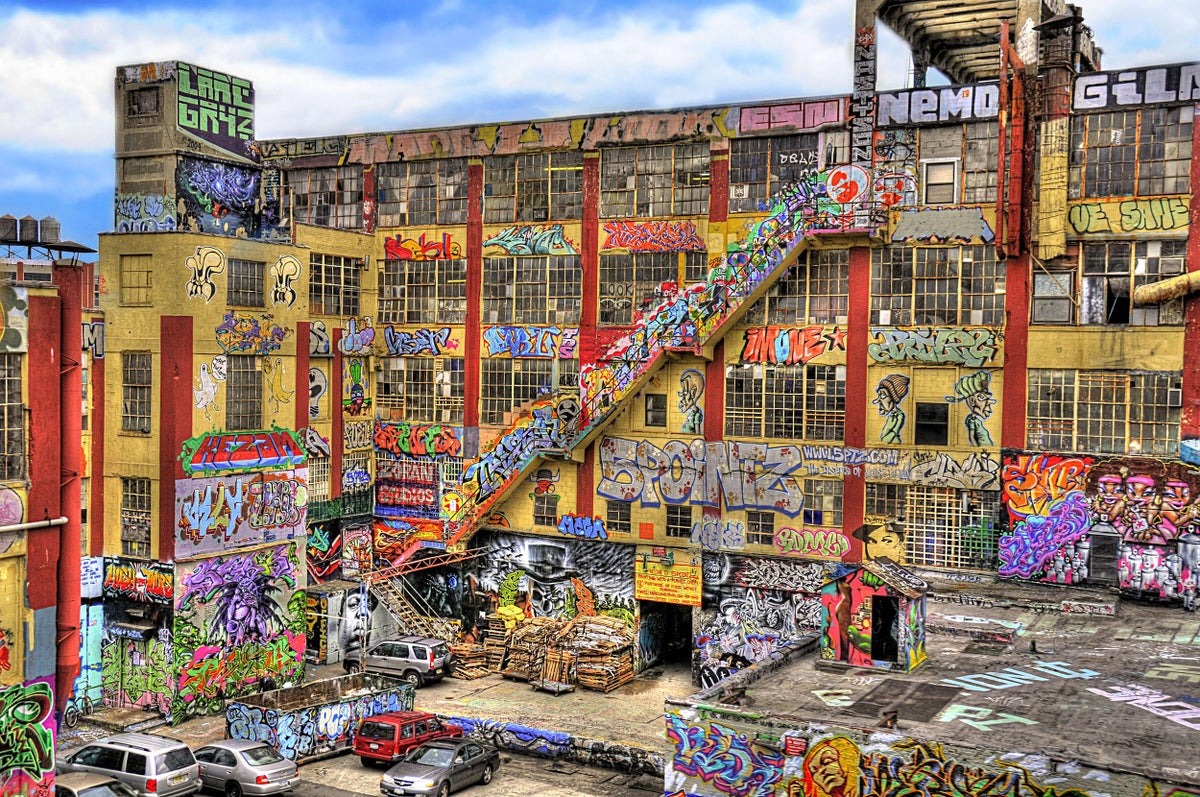This outdoor photograph showcases a massive, five-story building known as Five Points, formerly located in Queens. The structure is heavily adorned with graffiti, covering a significant portion of its facade, including a prominent staircase that ascends from the bottom left corner to the upper right section. The building, possibly an old warehouse or factory, features evenly spaced red columns that stretch from the ground to the top floor, interspersed with a grid of small square windows on nearly every level. Notable street art includes a variety of vivid murals, such as a sci-fi creature, a gold portrait of a man with dreadlocks surrounded by colorful paint, a skull wearing a top hat, and a portrait of Biggie Smalls. The name "Five Points" is boldly painted at the bottom center of the building. Adjacent to this main structure are several other buildings, and directly below, a parking lot filled with a mix of SUVs and compact cars.